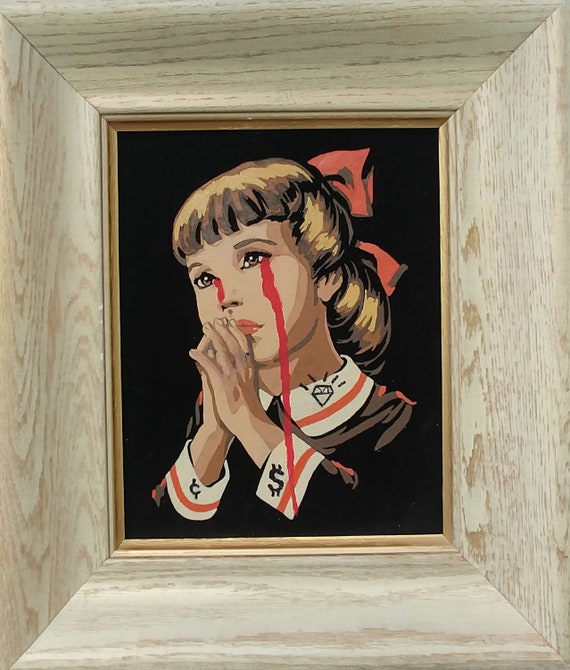The framed artwork displays a deeply evocative scene captured in a rectangular painting encased by an intricate white and light brown wood frame. The frame itself curves slightly outward, adorned with a visible wood grain pattern and subtle gold trim along its inner edge. The background of the image is in stark black, providing a striking contrast that draws the viewer's attention to the central figure—a young Caucasian girl with sharp bangs and long, curly blonde hair pulled back into a ponytail, tied with a bold red bow.

The girl's expression is one of somber intensity as she clasps her hands together in a prayer-like pose near her mouth. Her face shows red rivulets, suggesting tears of blood streaming down her cheeks and extending past her chin. She is dressed in a black top, accented by a stark white collar featuring a red stripe and an intricate diamond design in black lines, symbolizing value or worth.

Further reflecting themes of monetary value, the girl’s white cuffs mirror her collar design with red stripes. One cuff bears a cent symbol (¢), and the other displays a dollar symbol ($), perhaps making a poignant statement about greed, capitalist values, or the commodification of innocence. The use of colors—black, white, brown, red, pink, and yellow—enhances the depth and complexity of the message conveyed by the painting, possibly commenting on darker societal issues such as child labor or exploitation.